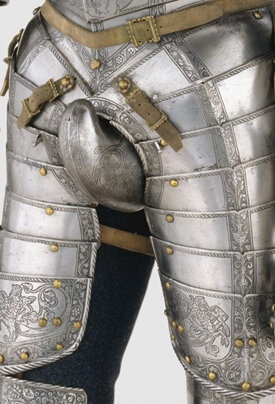The image showcases the lower half of a suit of armor, waist down to the knees, set against a light gray background visible at the bottom and in the upper left corner. The silver leg armor features horizontal grooves and gold studs along its borders, making it distinct and decorative. The design indicates that it’s composed of separate, interconnected pieces allowing movement. Above the waist, a tan leather belt with a brown metal buckle secures the armor, highlighting brown suede belt buckles on each side. Notably, there is a central, rounded, silver protective piece jutting outward, covering and safeguarding the groin area. The leg armor is attached to the front, hinting at black fabric underneath, suggesting the armor may be displayed on a mannequin. The lower edge, just above the knees, is richly engraved, enhancing its elaborate and historical appearance.